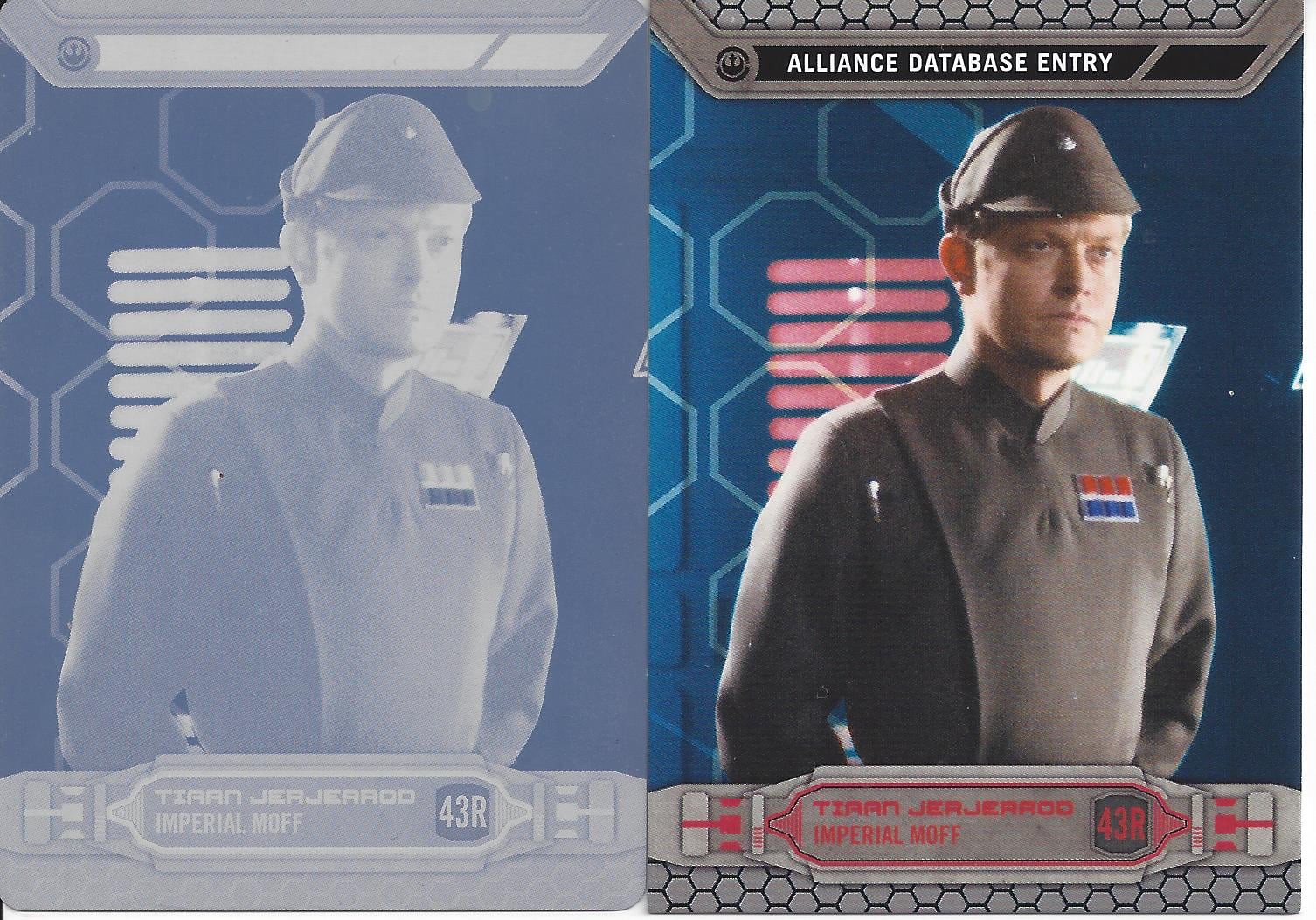The image is a split landscape orientation featuring two identical portraits side-by-side, resembling a pair of sci-fi trading cards. The right portrait is sharp and vibrant, while the left appears washed-out and foggy. Each portrait showcases a light-skinned man in a detailed, modern gray uniform with a rectangular badge bearing horizontal red, white, and blue stripes on his left chest. He is wearing a military-style cap. The clear image on the right reveals additional details: the top is labeled "Alliance Database Entry" in white letters on a black background, and beneath the man, in red lettering, is "Tyranjerico Imperial Moff 43R." The background has a blue hue with pink lines, enhancing its sci-fi aesthetic. The image combines elements of photographic detail, graphic design, and illustration, giving it the feel of a futuristic officer's card.